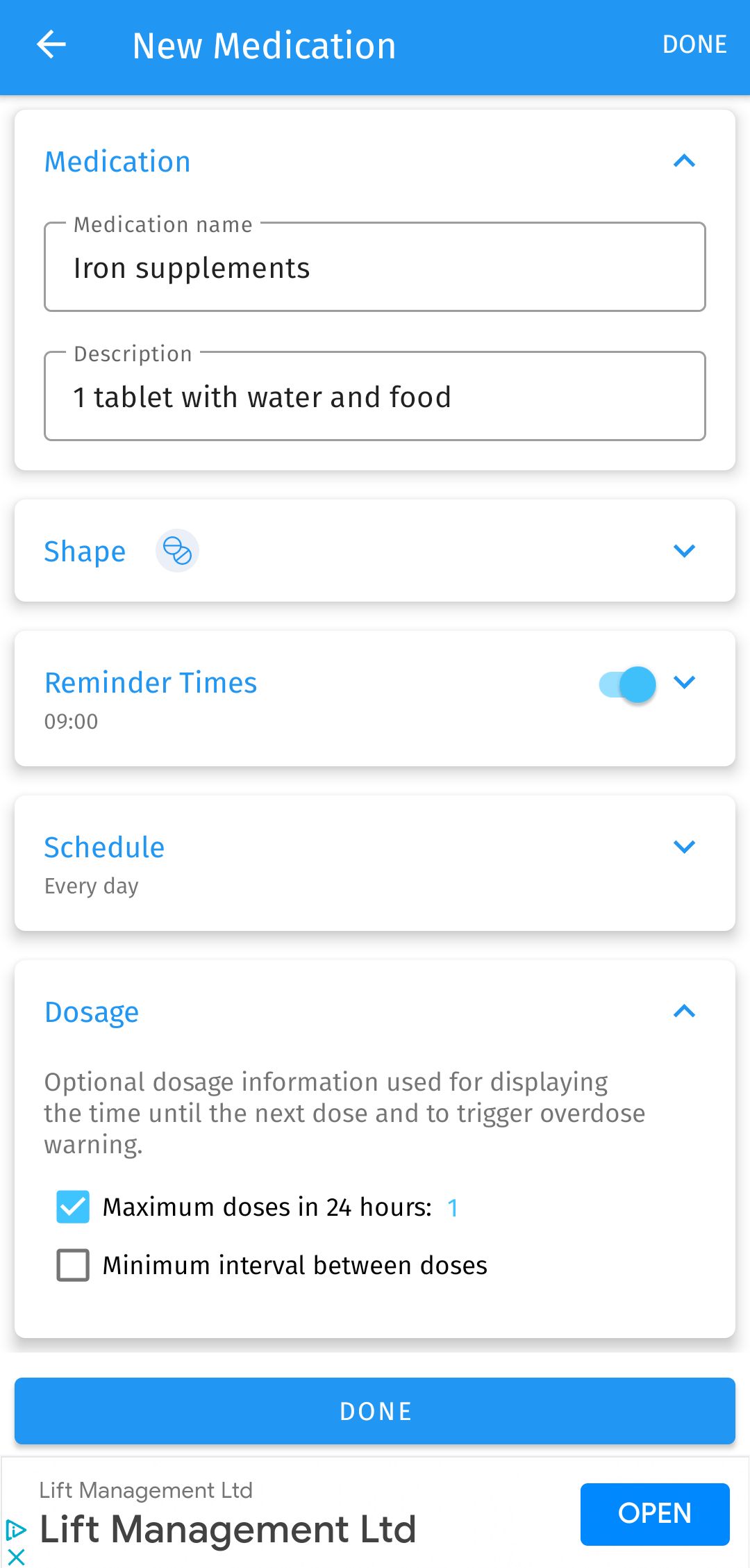The image features a clean white background, with a prominent blue rectangular box at the top. Inside this top box, there is a left-pointing arrow along with the labels "New Medication" and "Done," all rendered in white text. Below it, a rectangular outline in blue contains several sub-boxes and text entries: 

- A box labeled "Medication Name" contains the text "Iron Supplements" followed by a description, "One tablet with water and food." This box also has an upward-pointing arrow positioned at the top right corner.
- Another section titled "Shape" includes a right-aligned downward-pointing arrow.
- Under "Reminder Times," the time "09:00" is noted, accompanied by a small blue toggle switch and a downward-pointing blue arrow. The text also reads "Schedule: Every Day" with another accompanying downward arrow.
- The "Dosage" box includes an upward arrow and details that describe optional dosage information used for displaying the time until the next dose and triggering overdose warnings.
- There's a section with a blue check mark labeled "Maximum Doses in 24 Hours," followed by a smaller black box stating "Minimum Interval Between Doses."

Towards the bottom, there is a blue button labeled "Done," followed by a larger white box which includes a small right-pointing blue arrow with the text "Lift Management Limited" and another blue button labeled "Open." Finally, there's a small blue 'X' in one corner of the image.